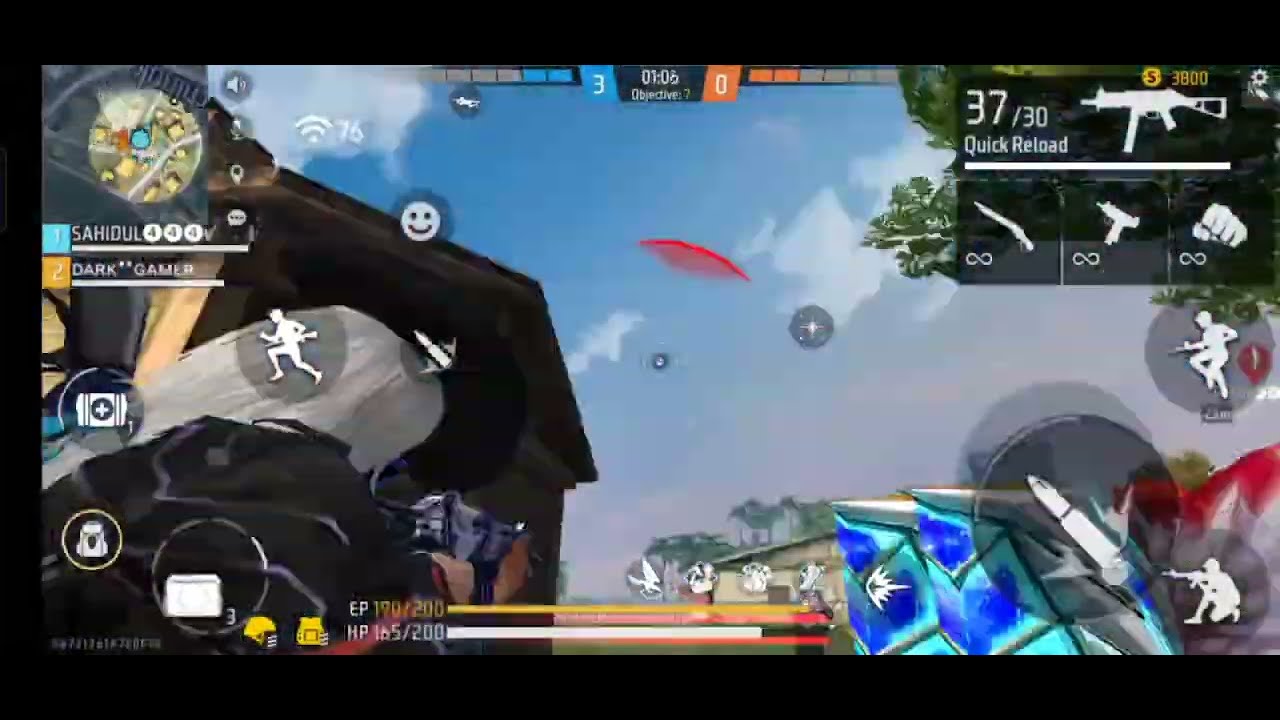This image is a slightly blurry screenshot from a video game, dominated by a detailed heads-up display (HUD) and an expansive sky view. The sky features mostly white clouds with a strip of blue, and prominently displays a paraglider with a red glider canopy. A character with silver hair and a black outfit appears in the bottom left corner of the screen. The edges of the screenshot are bordered by thin black rectangles at the upper, left, and bottom sides.

HUD elements heavily populate the screen edges: the upper right corner showcases various weapon icons, including machine guns, rifles, and an emoticon of a white fist, also displaying "37 / 30 Quick Reload." Different indicators and icons fill the lower right corner, featuring figures in various action poses with rifles, and geometric shapes in blue, teal, and red. The upper left contains a map, while the top center features progress bars showing values like 3, 0, and 0.1.